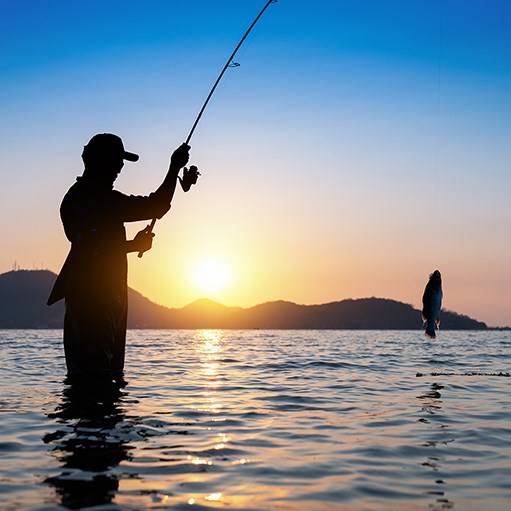In this outdoor photograph, we see a fisherman standing knee-deep in a large body of water, silhouetted against a stunning backdrop. The bright blue sky above transitions to a warm gradient of yellow and orange near the horizon, indicating either a sunrise or sunset. Far in the distance, the dark silhouettes of mountains or hills add depth to the scenery. The fisherman, also in silhouette, is wearing a shirt and a cap, with his fishing rod held vertically as he pulls a fish from the water. The fish, suspended on the far right side of the image, is clearly visible, dangling from the fishing line above the water’s rippling surface, which beautifully reflects the sun’s glow. The overall image captures the serene and picturesque moment with crisp clarity and natural lighting.